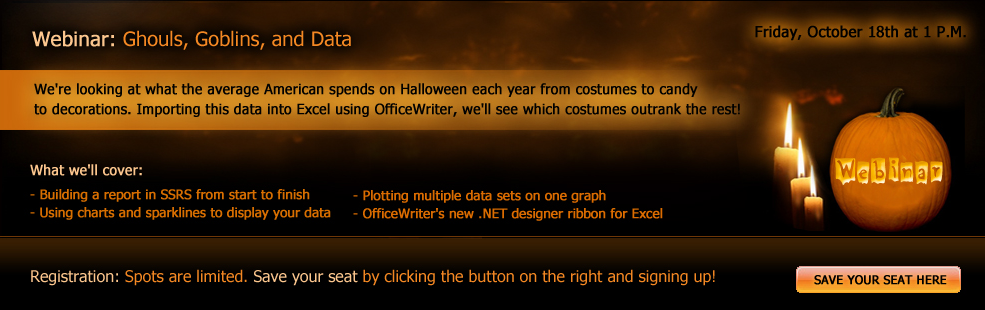### Detailed Caption for the Halloween-themed Webinar Screenshot

The image is a vibrant Halloween-themed webinar invitation presented in portrait mode, with a predominantly dark orange-brown background that sets the spooky tone. The upper left-hand corner prominently displays the word "Webinar" in white, followed by a bold, bright orange title: "Ghouls, Goblins, and Data." To the upper right, there is a section with an orange gradient background, announcing the date and time of the event: "Friday, October 18th at 1 p.m."

Beneath this, across the full width of the image, there's an expansive orange banner detailing the main focus of the webinar: "We're looking at what the average American spends on Halloween each year—from costumes to candy to decorations. Importing this data into Excel using Office Writer, we'll see what costumes outrank the rest." This informative banner sets the stage for the webinar's content.

Following the main theme, the next section outlines the agenda in an orange box: "What We'll Cover." The key points listed are:
- Building a report in SSRS from start to finish
- Using charts and sparklines to display your data
- Plotting multiple data sets on one graph
- Office Writer's new .NET Design Ribbon for Excel

To the right of this text, there's a visually engaging image of three vertically aligned, lit candles with high flames, enhancing the Halloween atmosphere. Adjacent to the candles, there is a carved pumpkin with its stem pointing to the right, and the word "Webinar" appears etched into the pumpkin.

At the very bottom of the image, a brown background carries a crucial call to action: "Registration spots are limited," emphasized with an orange highlight. This is followed by instructions in orange: "Save your seat by clicking the button on the right and signing up." The bottom right corner features an eye-catching orange button labeled "Save Your Seat Here," inviting viewers to register for the event. This clearly structured layout makes it evident that the image serves as an engaging and informative invitation to a Halloween-themed data webinar.